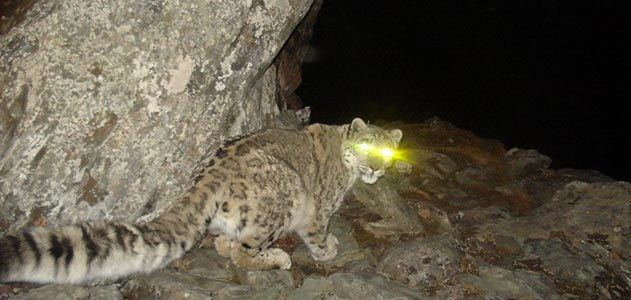The image captures a striking nighttime scene of a large wild cat, likely a mountain lion or bobcat, poised outdoors in a rocky, mountainous region. The cat’s light brown fur, with faintly visible patterns, shimmers under the minimal light, while its long, furry tail trails off to the left side of the frame. The animal is crouched on what appears to be a large rock or cliff, perhaps startled or lying low, gazing directly at the camera with eyes illuminated in a bright, eerie yellow by the camera's flash. The background to the top right is pitch black, accentuating the solitary and perhaps ominous presence of the cat, set against a backdrop of gray, sandy-colored rocks and a formidable boulder behind it. This photograph, seemingly captured by a stealthy wildlife photographer, conveys the raw and wild essence of nocturnal nature.